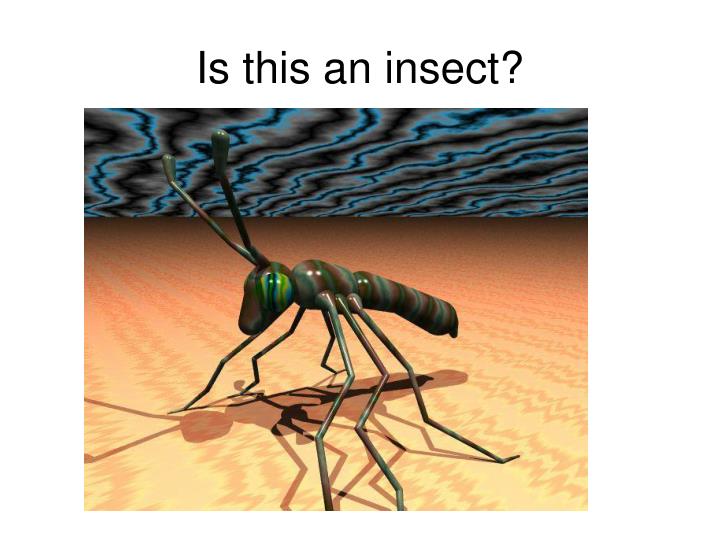Title: Is This an Insect?

Caption: The image features a cartoon-like model of a peculiar ant-like insect facing left. The ant, constructed from what appears to be light crystal or hard plastic material, showcases two long antennae and six legs. Its body is distinguished by brown and green striped patterns, which also adorn its elongated face. It stands on a yellow, sandy ground with wavy brown patterns, creating a striking shadow. Above the insect, the sky exhibits a marbled, wavy pattern in black, red, blue, and gray, reminiscent of electricity streaks. The foreground of the sand is significantly brighter, fading into darkness as it reaches the high horizon line that consumes the bottom two-thirds of the image. The black text at the top of the image reads, "Is this an insect?" adding a humorous, meme-like touch to the depiction.